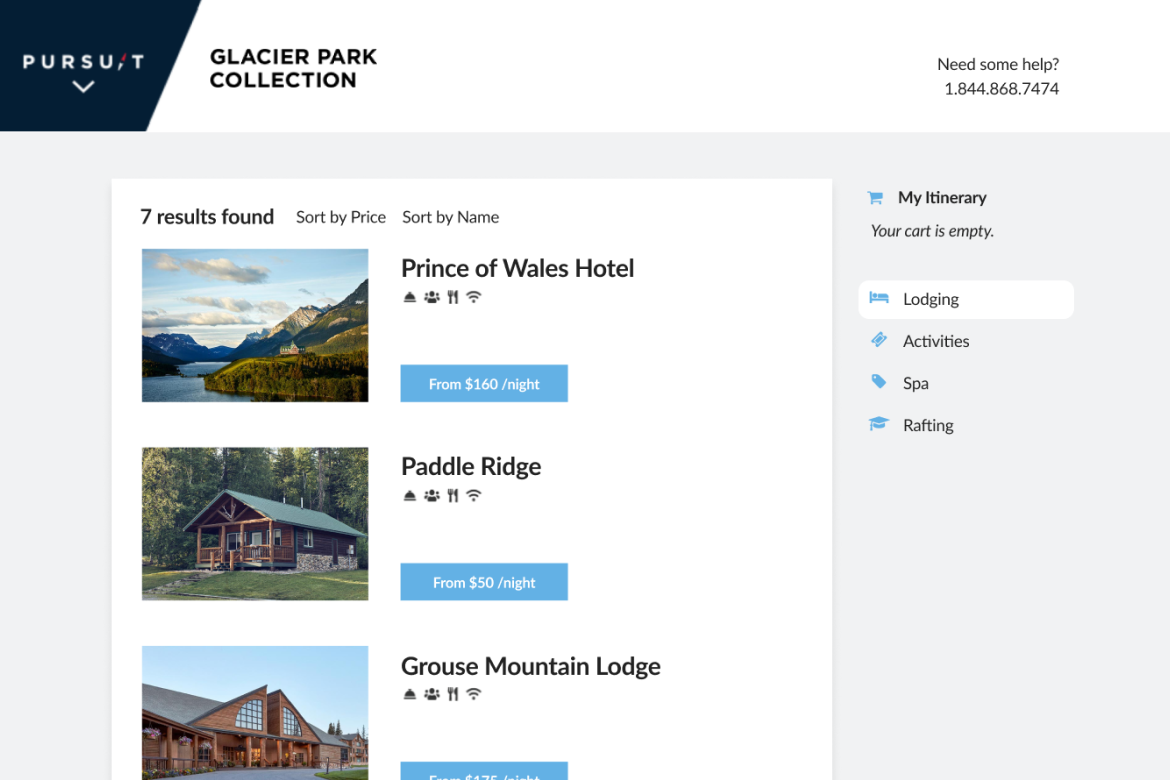The image depicts a section of the Pursuit website. At the top, the logo "PURSUIT" is prominently displayed with stylistic features: the "I" appears tilted and has pointed ends at the top and bottom, with the top half in red and the bottom half in white. Below the logo is a downward-pointing arrow, possibly indicating a dropdown menu, set against a background that appears to be either black or dark blue. 

To the right, the banner transitions to a white background featuring bold black text that reads "Glacier Park Collection". Adjacent to this, the text "Need Some Help?" is displayed alongside a phone number, 1-844-868-7474.

The next section of the webpage has a grayish background overlaid with three images. A bold caption in the top-left corner reads “Seven Results Found.” On the right, there are options to sort the results by price or name. 

The first image on the left features a serene scene of mountains, a body of water, and clouds, suggesting it was taken during the daytime. To the right of this image is the label "Prince of Wales Hotel", and beneath it, a price is displayed in a rectangle stating "from $160 a night".

Below this, an image labeled "Paddle Ridge" is shown, with a price listed as "from $50 a night."

Continuing downward, the "Grouse Mountain Lodge" (spelled G-R-O-U-S-E) is mentioned, but the price associated with it is cut off and not fully visible.